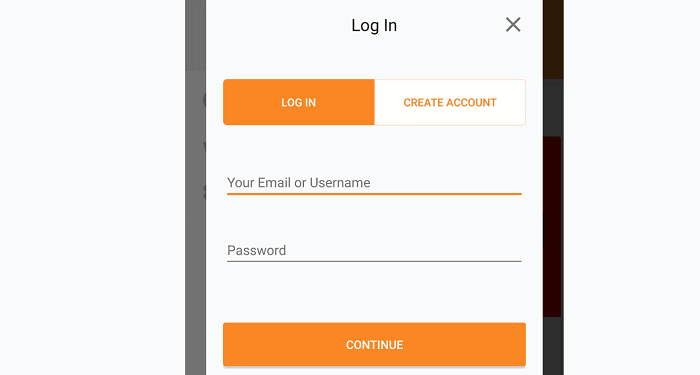The image displays a modern login landing page with a minimalist design featuring prominent black vertical bars on both the left and right sides. These bars enclose the main login interface, leaving blank space on their outer sides.

At the top center of the page, within the two black bars, the word "LOGIN" is displayed in all caps as two separate words. To the right of "LOGIN" is a small "X" icon, which serves as a button to close the login section.

Directly below this header, there is a significant blank space followed by a large horizontal rectangle that spans nearly the entire width of the screen. This rectangle is divided evenly into two sections: the left side is orange and contains the text "LOGIN" in white, while the right side is white with the text "CREATE ACCOUNT" in orange. Both texts are in all caps and displayed within a thin border outlining the rectangle.

Further down the page, a thin orange horizontal line stretches across the screen, immediately above which the text "Your email or username" is displayed, indicating where users should enter their credentials. Below this line, more blank space exists, leading to a gray horizontal line labeled "Password" in smaller, subtler text.

Towards the bottom of the page, there is a long orange button with white, all-caps text that says "CONTINUE." This button matches the length of the earlier divided rectangle for "LOGIN" and "CREATE ACCOUNT," emphasizing its importance as the final action for proceeding with the login process.